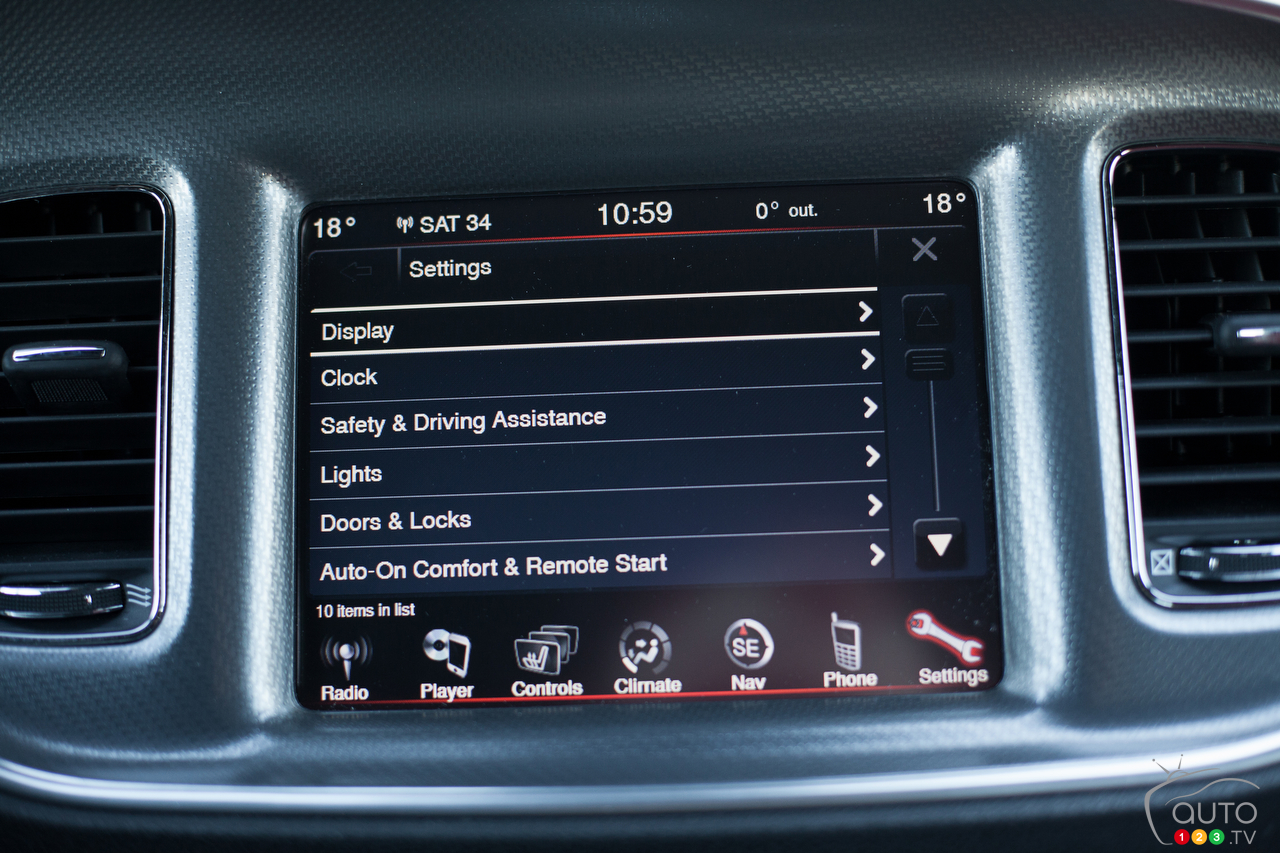The image showcases a close-up of the front dashboard of a newer model car, particularly focusing on the sophisticated user interface embedded in it. The dashboard is predominantly blue and gray, flanked by air conditioning and heat vents on both sides. The center of the display reveals a variety of control options and detailed information.

At the top, it shows the time, temperature, and various status indicators, including "18 degrees," "Sat," "10:59," and "0 degrees out." The main content of the interface is on the settings page, listing detailed options such as display, clock, safety and driving assistance, lights, doors and locks, auto on, comfort, and remote start, each accompanied by arrows for further navigation.

Below the settings list, there is an indication that there are "10 items" in the list. At the bottom of the display, various icons with descriptors such as radio, player, controls, climate, nav, phone, and settings provide access to different functions of the car. Notably, the bottom right-hand corner features a watermark that says "auto123.tv" accompanied by a graphic with red, yellow, and green circles.